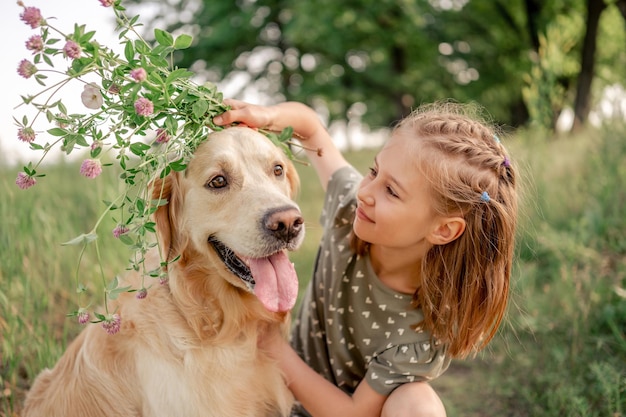The image is a professionally taken color photograph depicting a little girl and a golden retriever in a verdant outdoor setting. The girl is kneeling on a grassy path, bordered by tall green grass and surrounded by lush trees with medium-thickness brown trunks and abundant green leaves. Behind her, there is a field of what appears to be tall grass or wheat. She has light brown to blonde hair styled in French braids that flow down to her shoulders.

The girl is wearing an olive-green shirt adorned with small white flower and heart patterns. She is holding a bouquet of pink, red, and white flowers with some greenery, and is gently placing the flowers over the dog's head, her other hand resting on the dog's neck. The golden retriever, with its tongue hanging out, looks content as the girl gazes at it with a soft smile. The background is slightly blurred, emphasizing the intimate and tender moment between the girl and her dog. The overall color palette of the image is neutral, adding to its serene and natural feel.